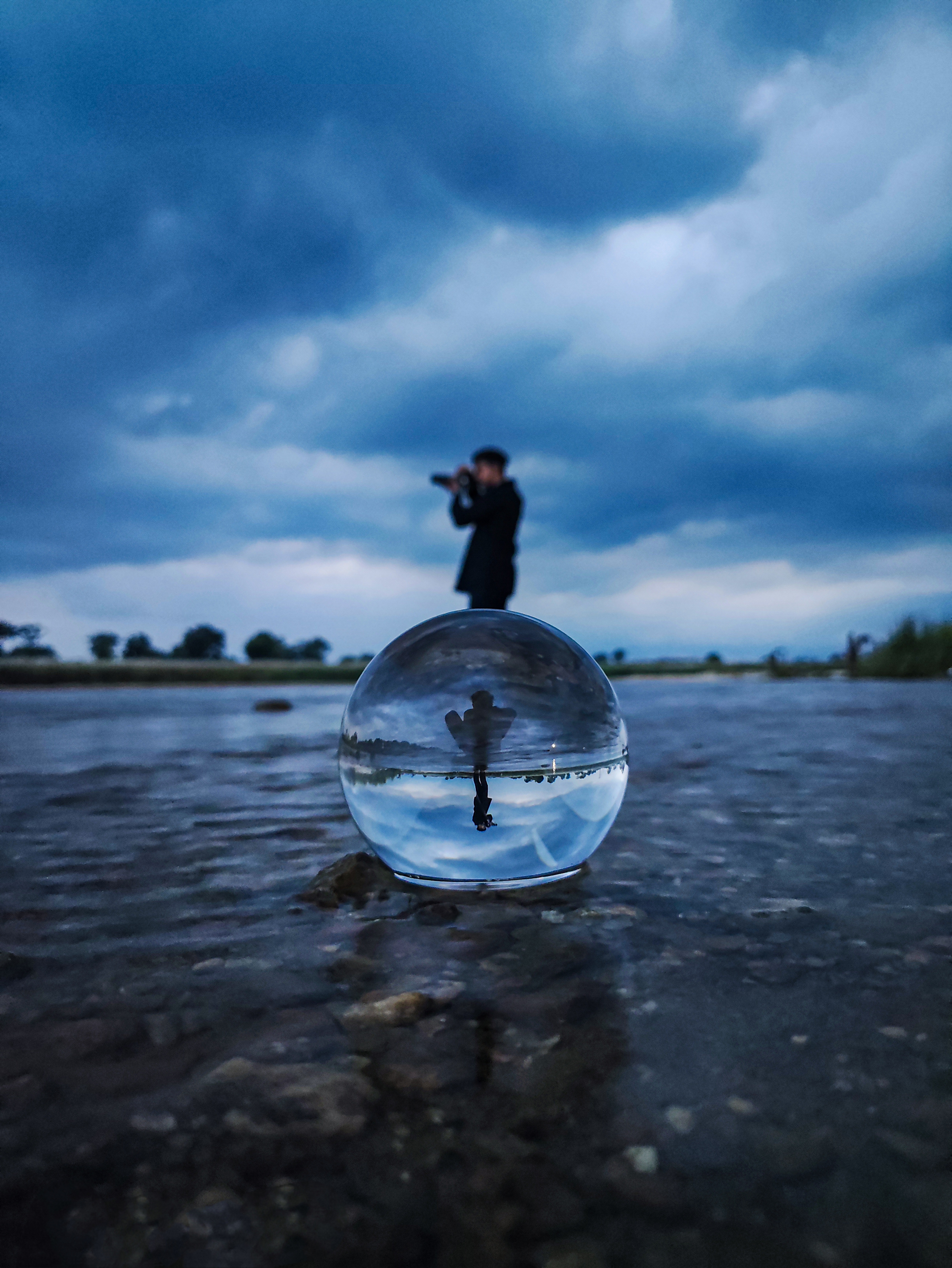In the photograph, a man stands in the center, waist-deep in a shallow, clear body of water. He wears a black coat and faces left, holding a camera poised to capture a scene off to that direction. The backdrop is characterized by a dark, moody sky with dense, overcast clouds, hinting at stormy weather, and a distant shoreline dotted with a few scattered trees.

In the foreground, atop the water's surface, rests a glass sphere resembling a snow globe. This orb refracts and reflects the scene around it, rendering an upside-down image of the man and the sky. Intriguingly, the sphere captures the man’s reflection within it, generating a visual effect where the man appears inverted in the sky above the water within the glass orb. The overall composition skillfully intertwines the elements of water, reflection, and the mysterious atmosphere of the approaching storm.